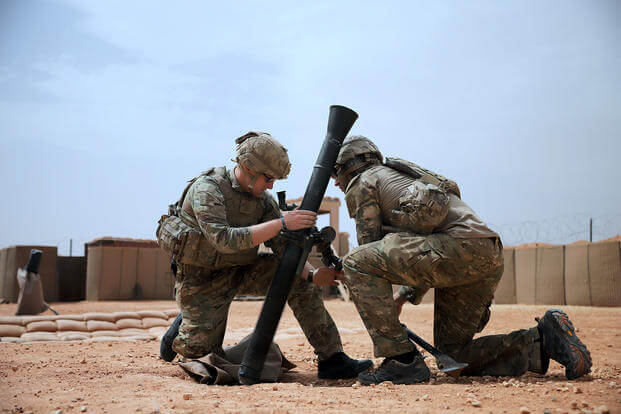In this image, two military soldiers are kneeling on a dirt surface, seemingly on a base or camp surrounded by sandbags and barriers topped with curled barbed wire. Both are dressed in full military gear, including urban-style camouflage uniforms, helmets, and goggles. They are intently examining or setting up a black, tube-like object, likely a missile launcher or bazooka, which they hold between them, pointed upward. The background showcases a cloudy blue sky that dominates a large portion of the scene, with sunlight breaking through, casting a contrast on the otherwise tense and focused atmosphere of the soldiers' task. No other individuals are present, emphasizing the concentration of these two men on their equipment and mission.